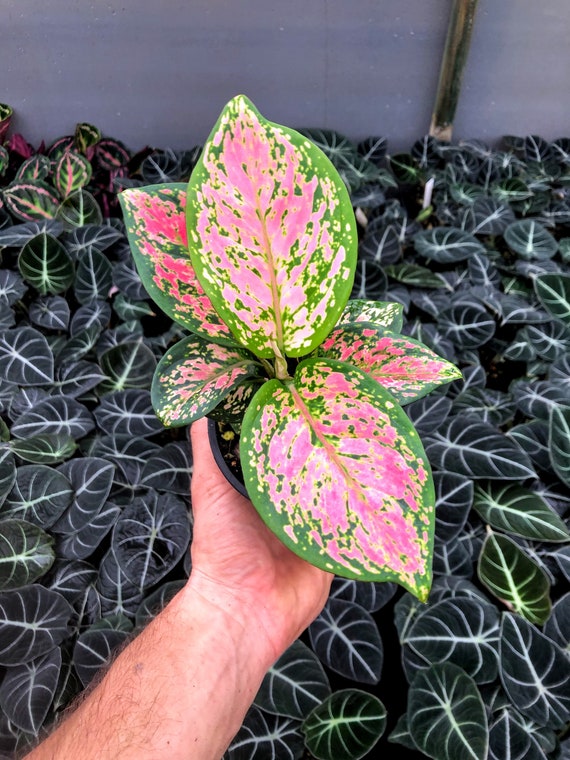This photograph showcases an outstretched, hairy man's arm emerging from the lower left corner, holding a flower pot with a caladium plant. The caladium features large, waxy leaves that are green with prominent pink markings. The pot, partially visible and appearing to be plastic with a black rim, is held securely in his hand. The camera angle looks down on the plant, giving a detailed overview of the vibrant foliage. Below the hand and pot, the background is filled with a dense arrangement of similar plants, possibly begonias or hostas, characterized by their dark green leaves and striking white veins. Amidst this verdant setting, a bluish-gray building and a gold post run up the right-hand side, adding structural elements to the scene. This detailed image captures the lush, varied textures and colors of the indoor plants against the subtle backdrop of the room.